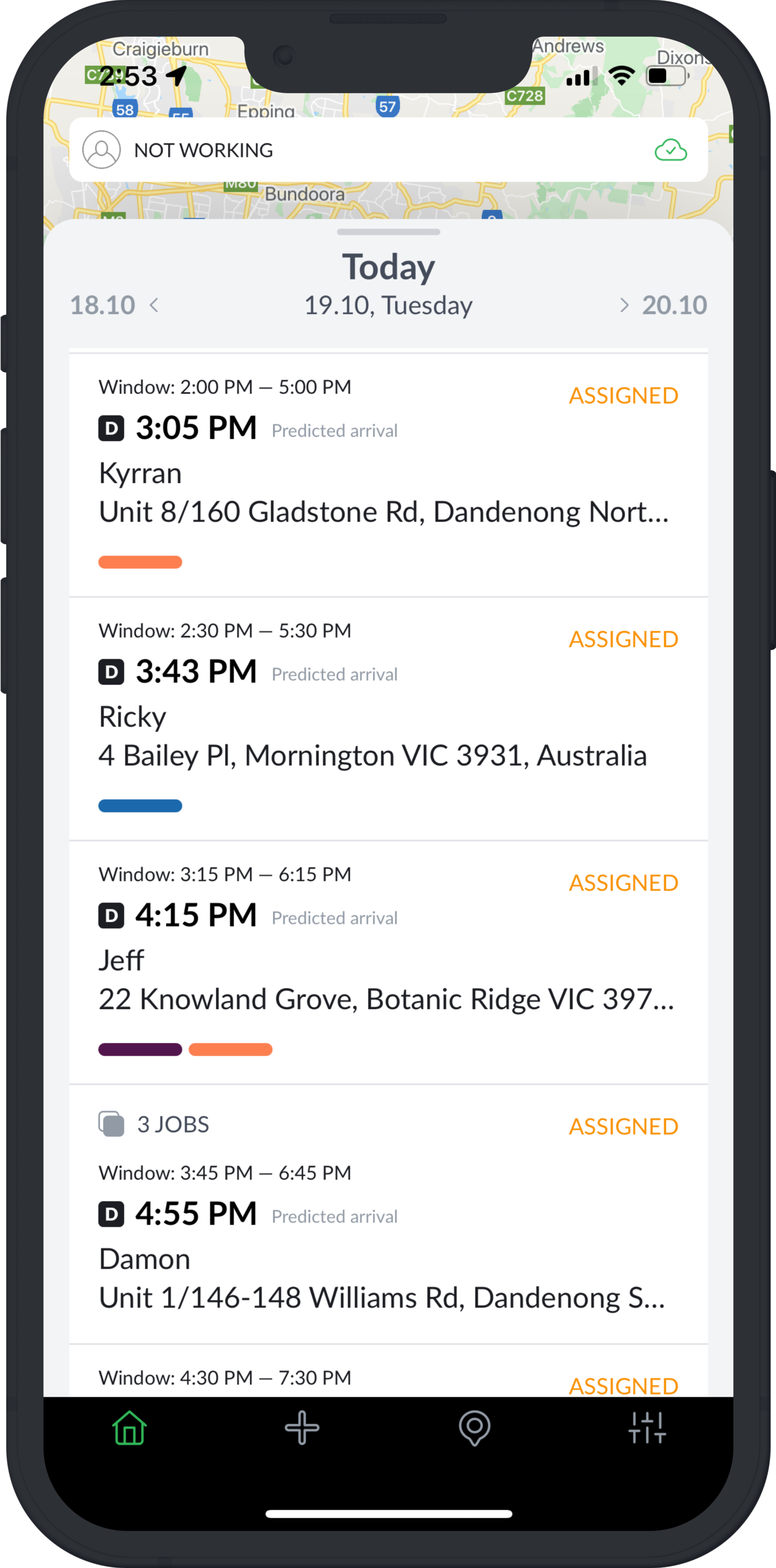The image depicts a smartphone, specifically styled like an iPhone, with a thin black outline. At the top of the phone screen, a map's background is visible. The screen displays several pieces of information in various sections. 

Starting from the top, the map highlights two locations: "Craigieburn" with "C R A I G I E B U R N" in capital letters, and "Andrews." The time is displayed as "2:53 PM" on the right side of the top bar alongside icons for battery level, Wi-Fi signal, and cell signal.

Beneath this, a banner in uppercase text reads "NOT WORKING." On the right side of this banner, there's an outlined green cloud with a green checkmark inside it. Below this banner, the background turns white with gray borders along the top and sides. It shows the dates "1810" and "2010," followed by "TODAY" and "19.10." with "Tuesday."

The screen is divided into four sections, each detailing different time windows for assignments:

1. The first section lists "Windows 2:00 PM to 5:00 PM" with an assigned time of "2:43 PM" for predicted arrival at Chiron Unit 8, located at 160 Glaston Road.
2. The second section shows a time window of "2:30 PM to 5:30 PM" and "2:43 PM" as the predicted arrival time. The assignee, Ricky, is scheduled for 4 Bailey MPL in Mornington, Vic, Australia.
3. The third section indicates a "3:15 PM to 6:15 PM" window with a predicted arrival of "4:15 PM." Jeff is assigned to 22 Nolan Grove in Botanic Ridge, Vic.
4. The final section lists "3:45 PM to 6:45 PM" with three jobs assigned for "4:55 PM," handled by Damon at Unit 1/146-148 Williams Drive.

Overall, the image organizes logistical details and schedules across different locations, displayed through a sleek smartphone interface.